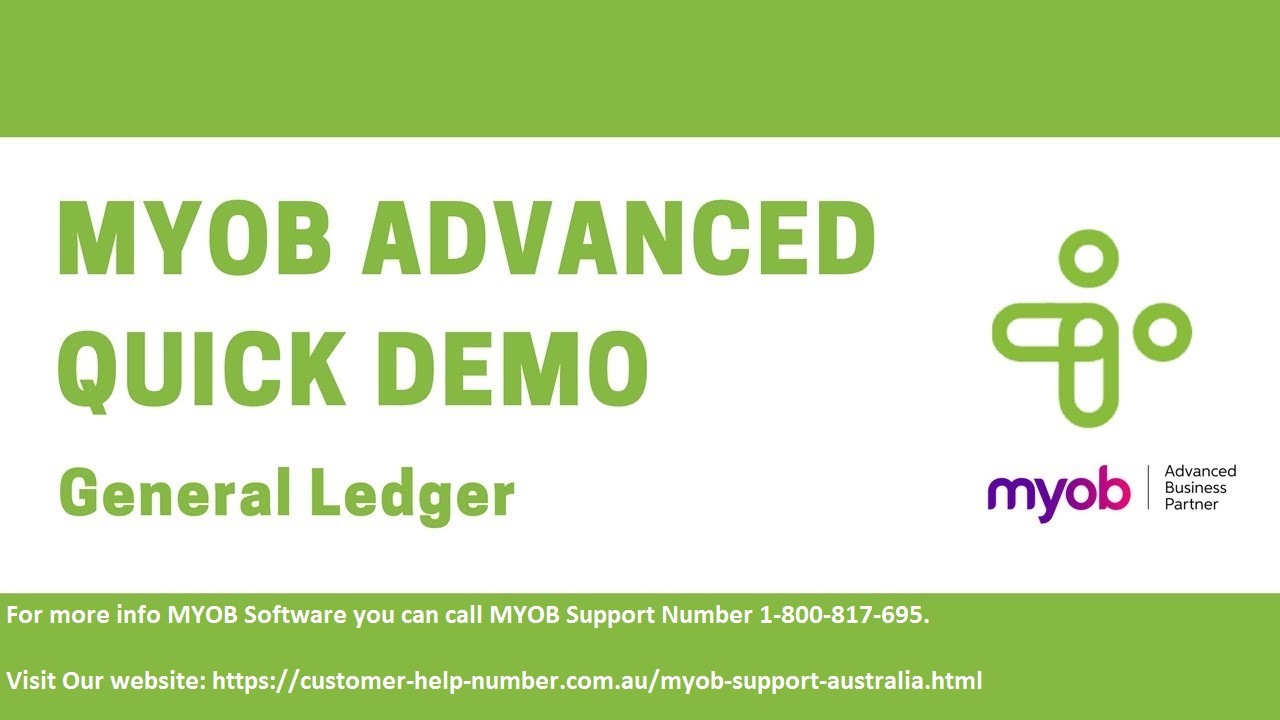The image is a promotional poster for MYOB accounting software, specifically highlighting the MYOB Advanced Quick Demo for the General Ledger. The layout features a green border on the top and bottom, with a white center section. The top green section is blank, while the center white area prominently displays the text "MYOB Advanced Quick Demo General Ledger" in green on the left side, and the MYOB logo on the right. The logo consists of two stylized 'I's, one normal and one with the dot positioned to the right. Below the logo, it states "MYOB Advanced Business Partner". The bottom green section provides contact information for further assistance, including the MYOB support phone number, 1-800-817-695, and a URL for their Australian support website: https://help-number.com.au/MYOB-support-australia.html.